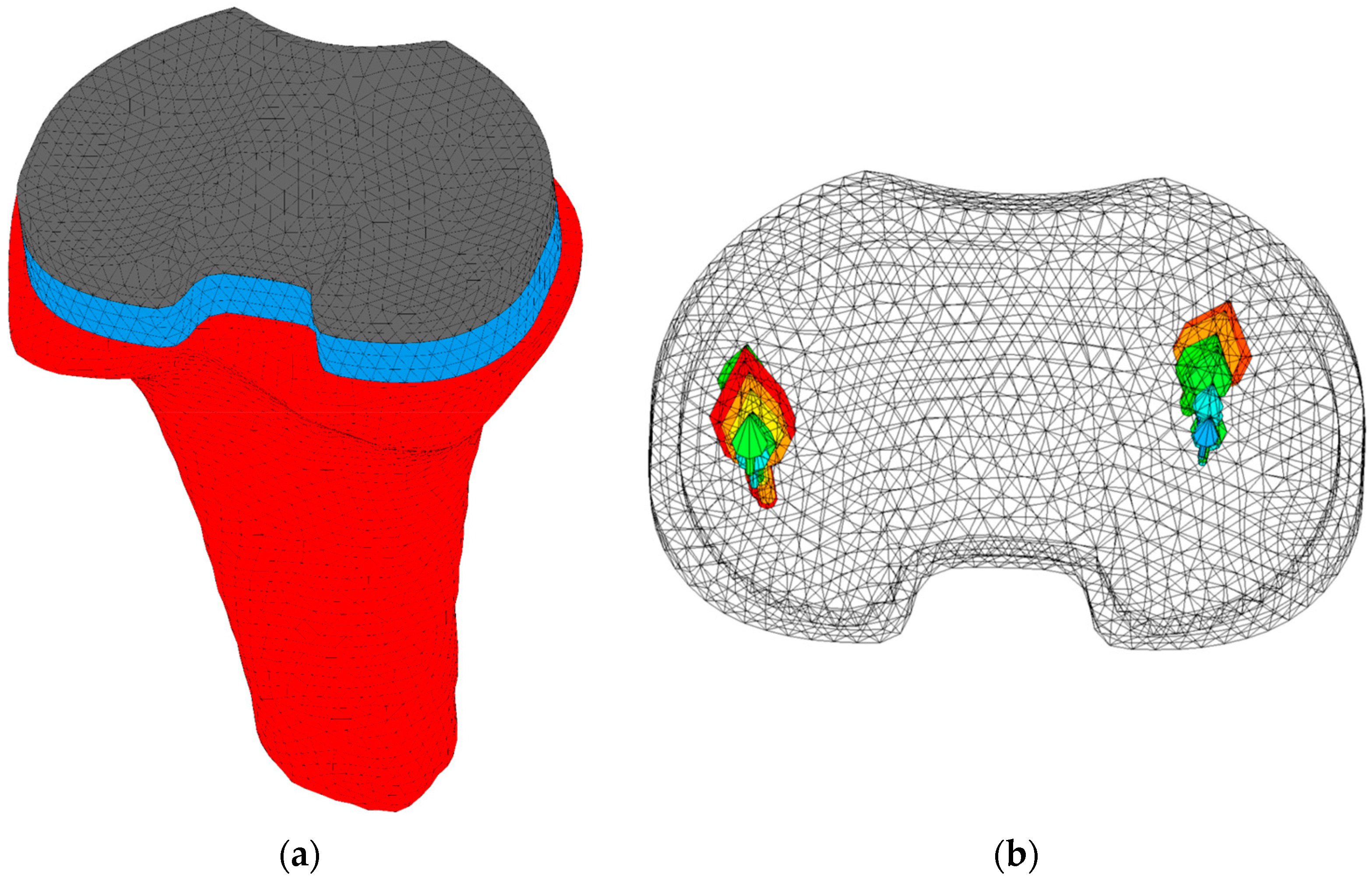This is a computer-generated rendering of two side-by-side stamps, labeled A and B. Image A features a stamp with a red handle pointing downward, revealing a blue, netted design on its bottom, resembling a Batman signal, with a dark gray top. Image B displays a diamond-textured pattern adorned with red, green, and blue stamps on either side, and has a colorful, game-controller-like design. Both images feature intricate 3D modeling line work that highlights the geometry of the forms.